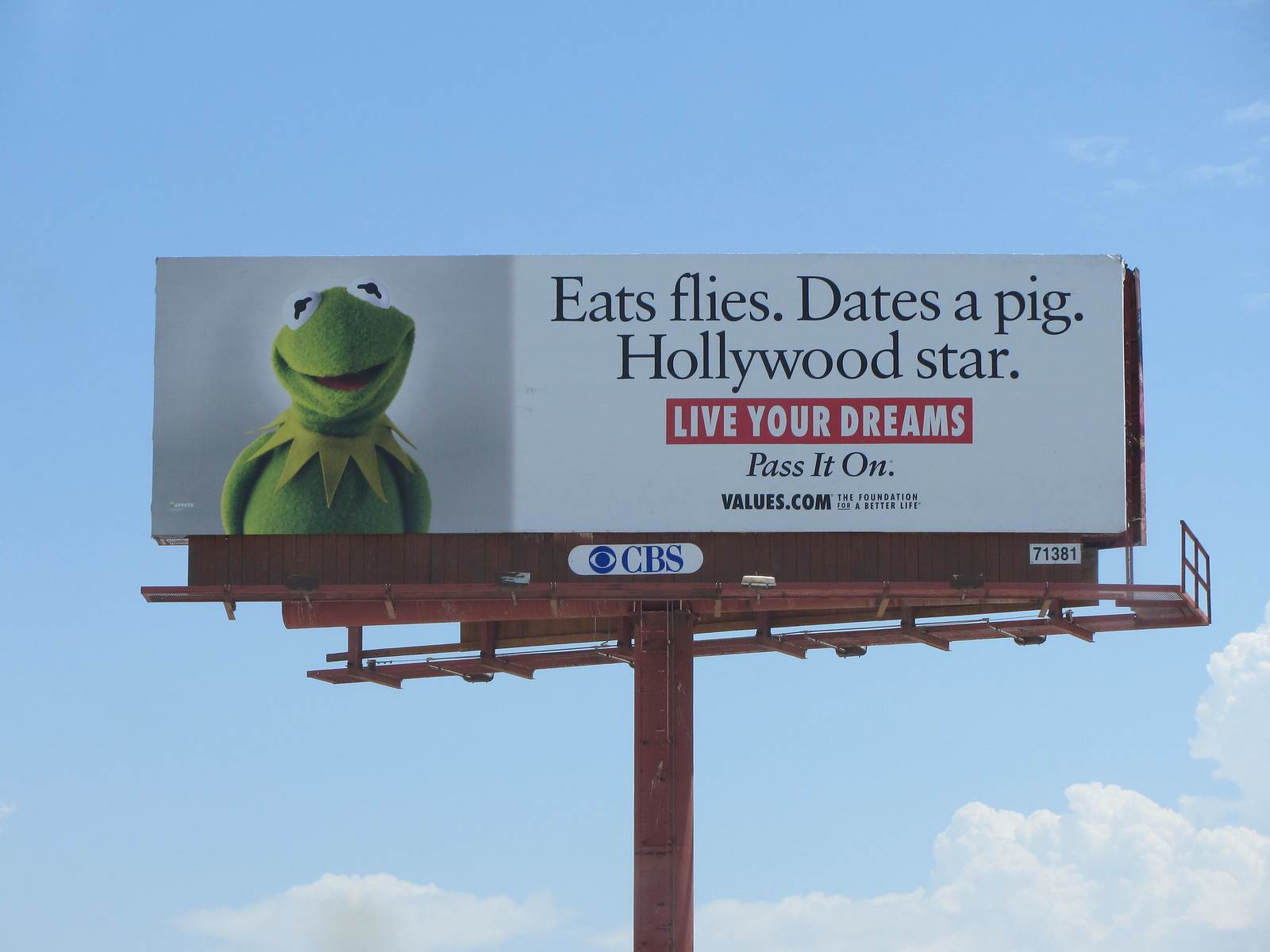The image depicts a roadside sign mounted on a pole, with a clear sky and a few clouds visible near the bottom of the frame, giving the impression that the photo is taken from a slightly low vantage point looking upward. The main feature of the sign is an image of Kermit the Frog set against a gray background, located on the left side of the sign. To the right of Kermit's picture, several statements in bold text proclaim: "Eats flies, dates a pig, Hollywood star." Below this, in striking red letters, the sign encourages passersby with the message, "Live your dreams." Further down, in smaller text, the sign credits "values.com" and prompts viewers to "pass it on." In the bottom right corner of the sign, the CBS logo and the letters "CBS" are clearly displayed, as well as a distinct number "71381" in white. The overall design of the sign conveys a motivational message, blending celebrity familiarity with an inspiring call to action.